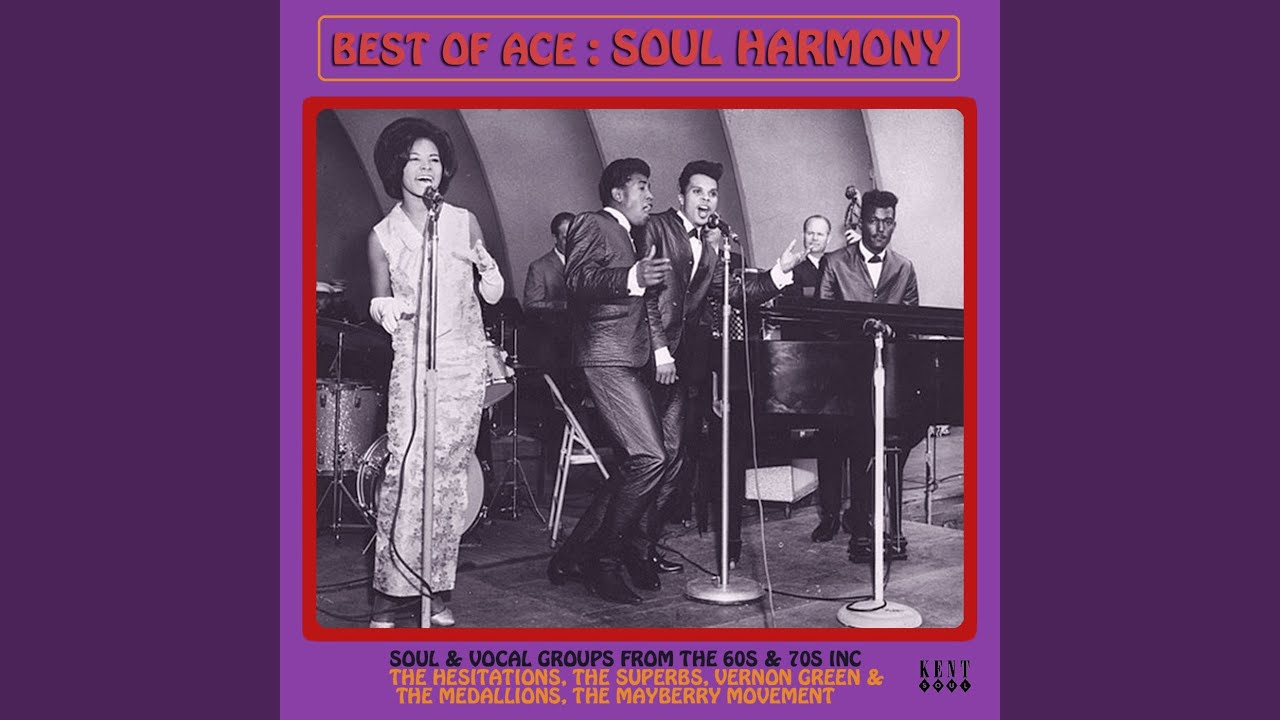The album cover is vintage, predominantly in shades of purple, bordered by a darker purple frame. "Best of Ace, Soul Harmony" is prominently displayed in red text at the top. The cover features a central, black-and-white photograph of a lively group of soul singers from the 60s or 70s, encapsulating the essence of that era. The image showcases six African-American performers: a woman singing into a microphone on the left, two men singing into another microphone in the middle, a man playing the piano on the right, a bassist in the background, and a sixth person partly visible behind the singers. Beneath the image, yellow text lists notable soul and vocal groups including The Hesitations, The Superbs, Vernon Green, The Medallions, and The Mayberry Movement, accompanied by a black label stating "Soul and Vocal Groups from the 60s and 70s, Inc." A logo, possibly from the record label Kent, is positioned at the bottom right corner. The overall design is set against a plain, lighter purple background, radiating a nostalgic charm of classic soul harmony.